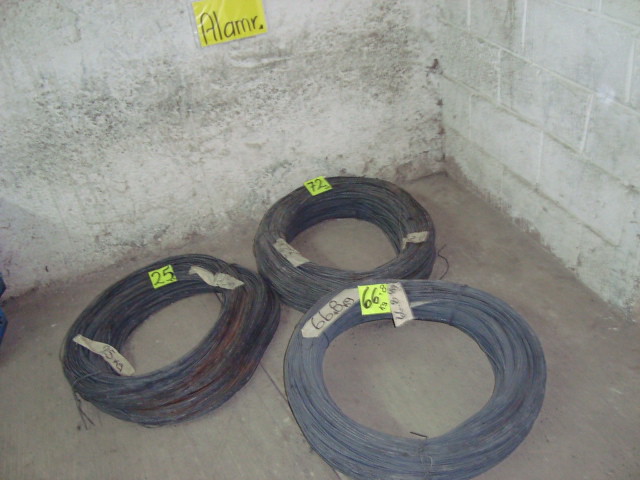A rather faded color photograph, square in format, appears to have been taken indoors. The scene features a light gray or white concrete block wall, which looks dirty and smudged. At the top of the wall, there is a yellow plastic sign with black handwritten lettering that spells "Alamar." The floor, which seems to be light brown or cement, showcases three very badly worn-out, rusted tires arranged in a triangular pattern. Each tire has a neon yellow-green post-it note with a number: 25 on the left tire, 72 on the top tire, and 66.8 on the bottom tire. Additionally, there is some brown tape with unreadable black handwritten numbers on it affixed to the tires.